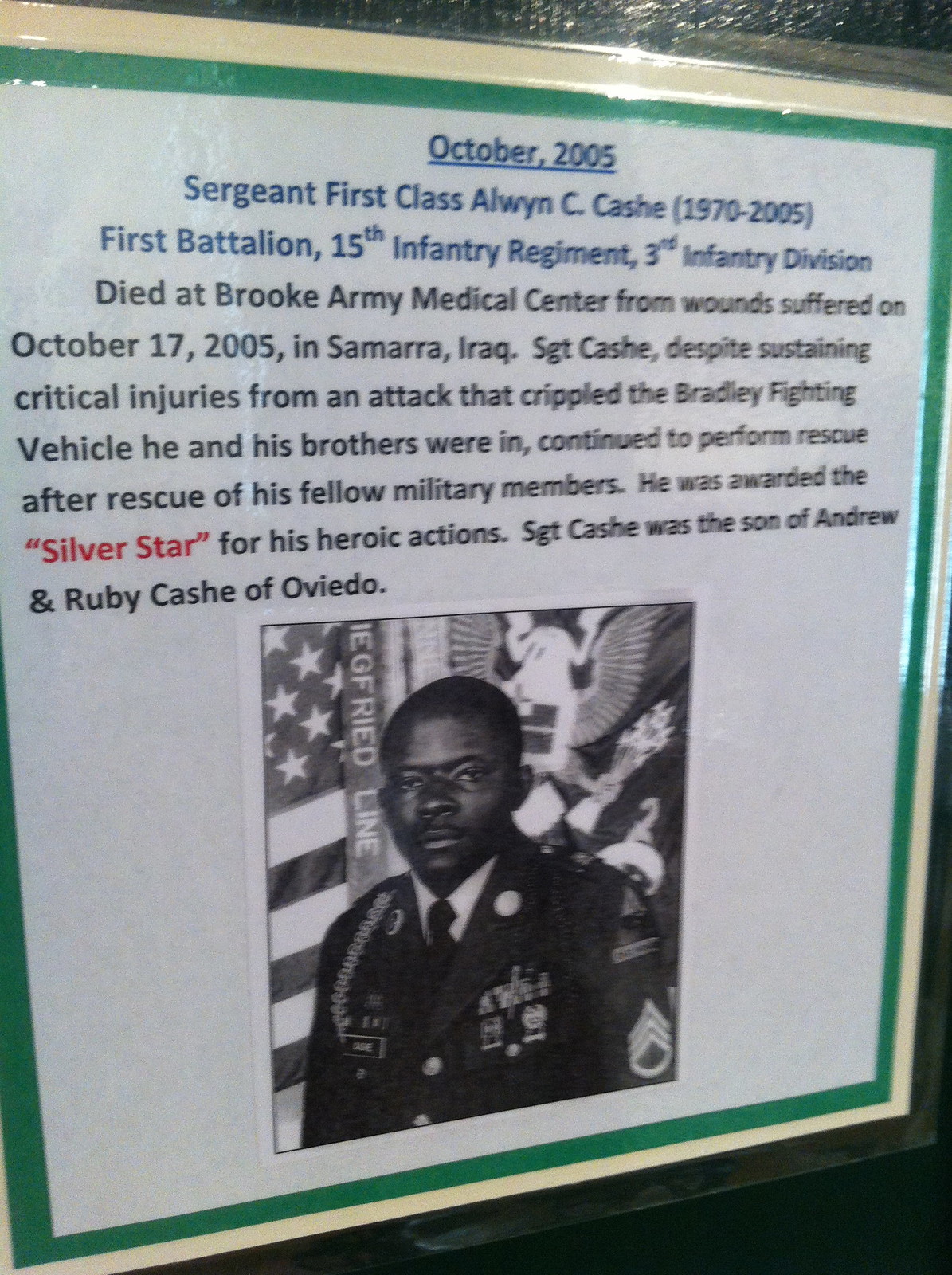The image depicts a laminated sign bordered in tan and green hues with an off-white interior. At the top, in blue ink, it reads: "October 2005, Sergeant 1st Class Alwyn C. Cash, 1970-2005, 1st Battalion, 15th Infantry Regiment, 3rd Infantry Division." Below the title is a black and white photograph of a young African American man in military uniform with the American flag and another flag in the background. The inscription, detailed in black ink, recounts the heroic actions of Sergeant Cash. It states he died at Brooke Army Medical Center from injuries sustained on October 17, 2005, in Samara, Iraq. Despite his critical injuries from an attack that damaged the Bradley Fighting Vehicle he was in, Sergeant Cash continued rescuing his fellow soldiers, actions for which he was awarded the Silver Star. The text also notes that Sergeant Cash was the son of Andrew and Ruby Cash of Oviedo.